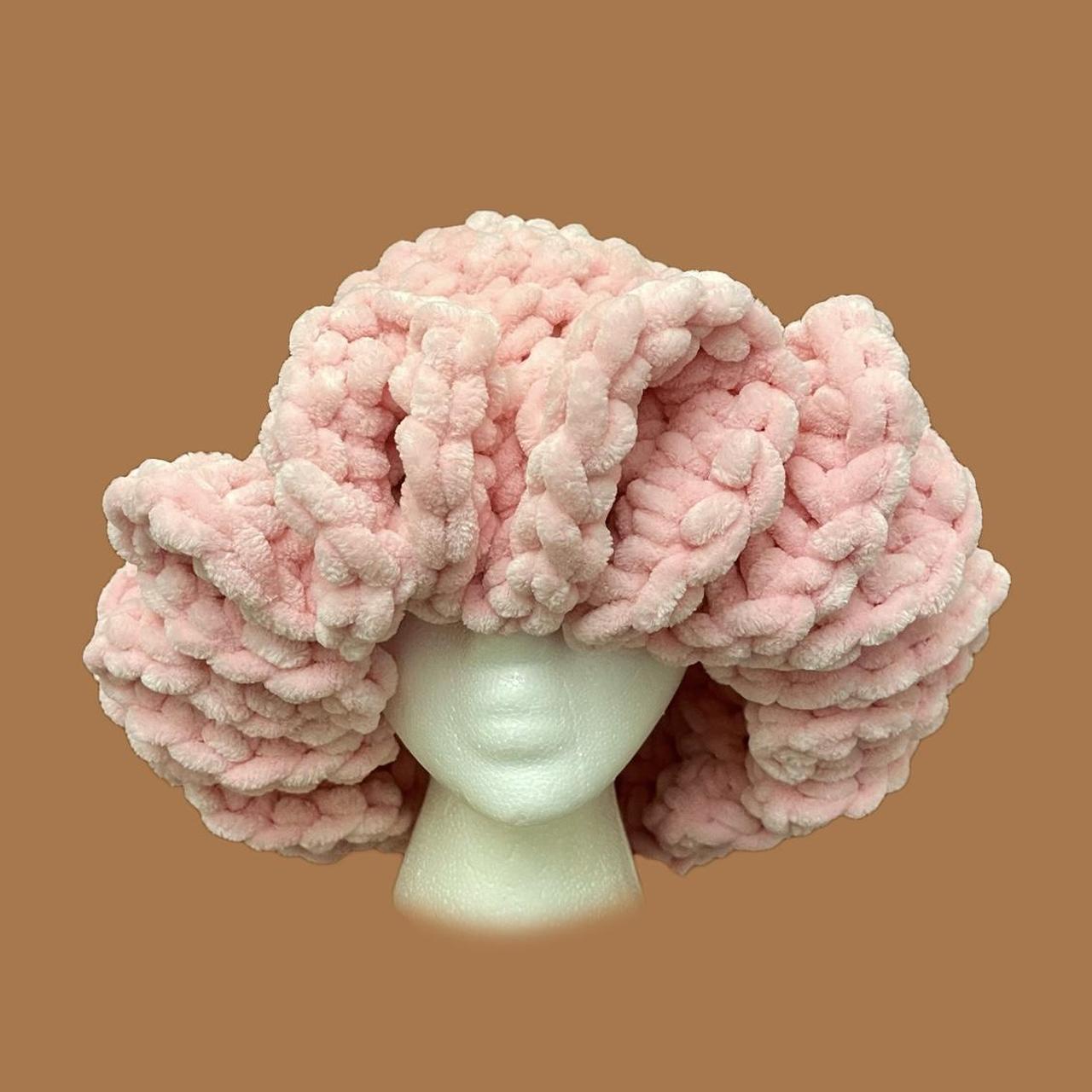The image showcases the bottom half of a styrofoam mannequin head, draped with a large, poofy pink hat. The hat, likely crocheted or knitted, is constructed from thick, fuzzy yarn reminiscent of the material used in baby blankets or resembling the woolly texture of a sheep. The hat extends around to the back of the head and features ruffled edges, while appearing more smooth on top. This scene is set against a brown gradient background, which transitions from a darker tone at the top to a lighter, tan and peach-colored hue at the bottom. The overall composition highlights the contrast between the soft, textured hat and the sleek, styrofoam mannequin head.